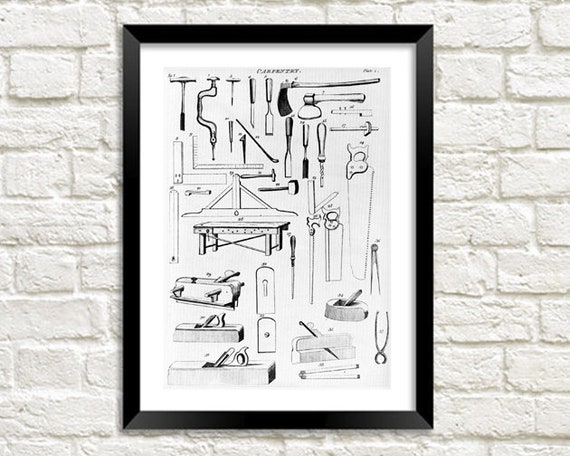The image features a white brick wall, heavily painted over time, serving as a backdrop for a piece of monochromatic artwork. Central to the image is a black-framed and white-matted piece of art, which appears to be a detailed pen and ink drawing on a gray background. The drawing illustrates an array of approximately 25 antique-style tools, meticulously sketched in black and white. The tools range from widely recognized items like saws, hammers, chisels, axes, screwdrivers, and levels, to more specialized and historical implements such as old-school drills and glass-holding tools. Arranged systematically, these tools lack individual labels, though some faint text, possibly reading "carpentry," is visible at the top. The overall composition exudes a modern aesthetic, suitable for display in a contemporary setting.